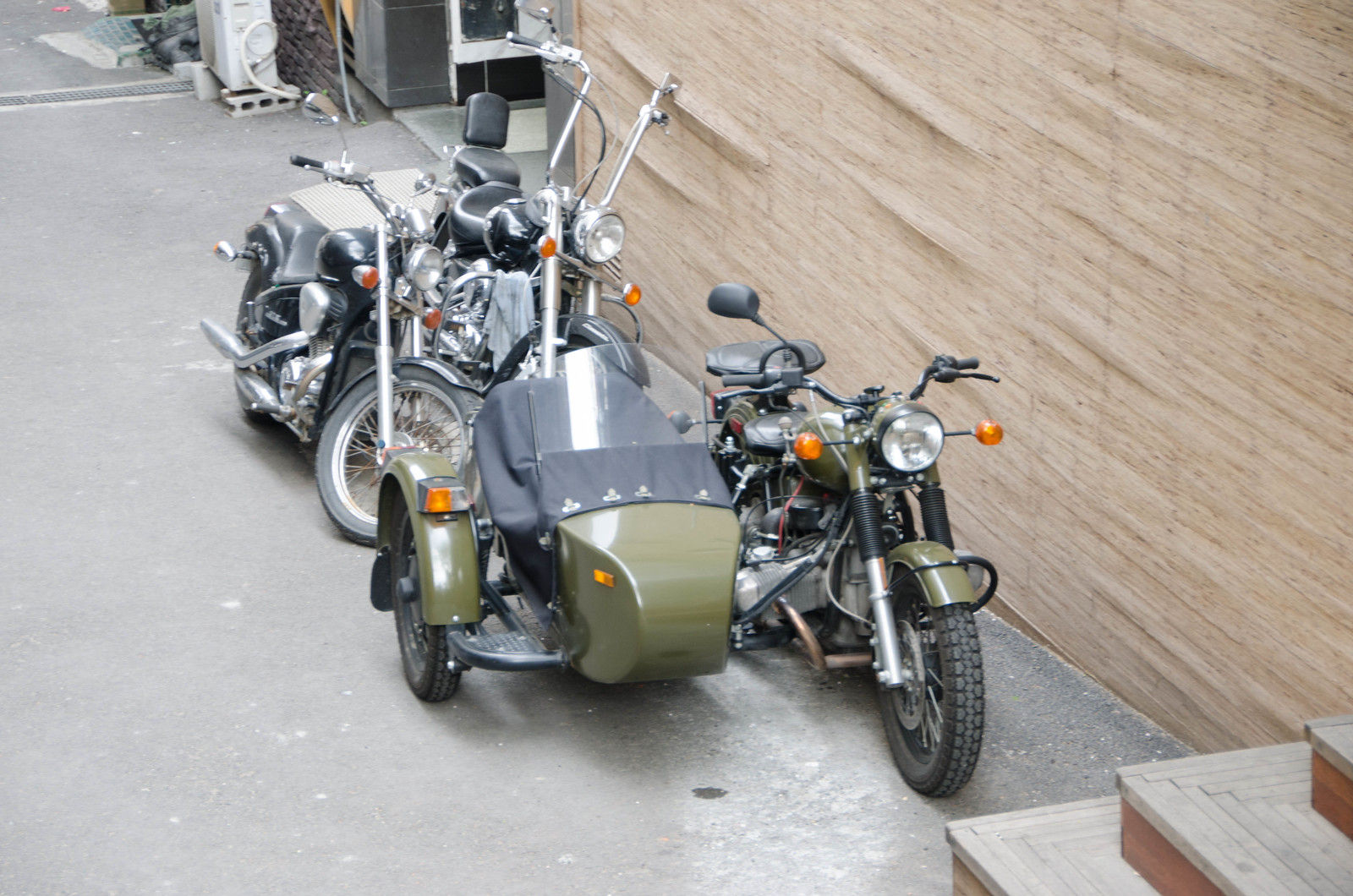The photograph depicts a parking area in front of what appears to be a building, featuring three distinct motorcycles. The central focus is a motorcycle with an olive green sidecar, accented with black and highlighted by a large front light. Positioned behind it is another motorcycle, elegant in chrome and gray tones, possibly sporting another sidecar or elaborate accessories. To its right stands a third motorcycle, black and sleek, equipped with a passenger seat. The scene is set against a pale beige wall resembling bamboo and a plain concrete driveway. Visible details include a short staircase at the lower right, what looks like some construction materials or garage items in the upper left, and a small oil stain on the ground near the green motorcycle. An opening leading into the building, along with some vent and pole-like structures, completes the backdrop.